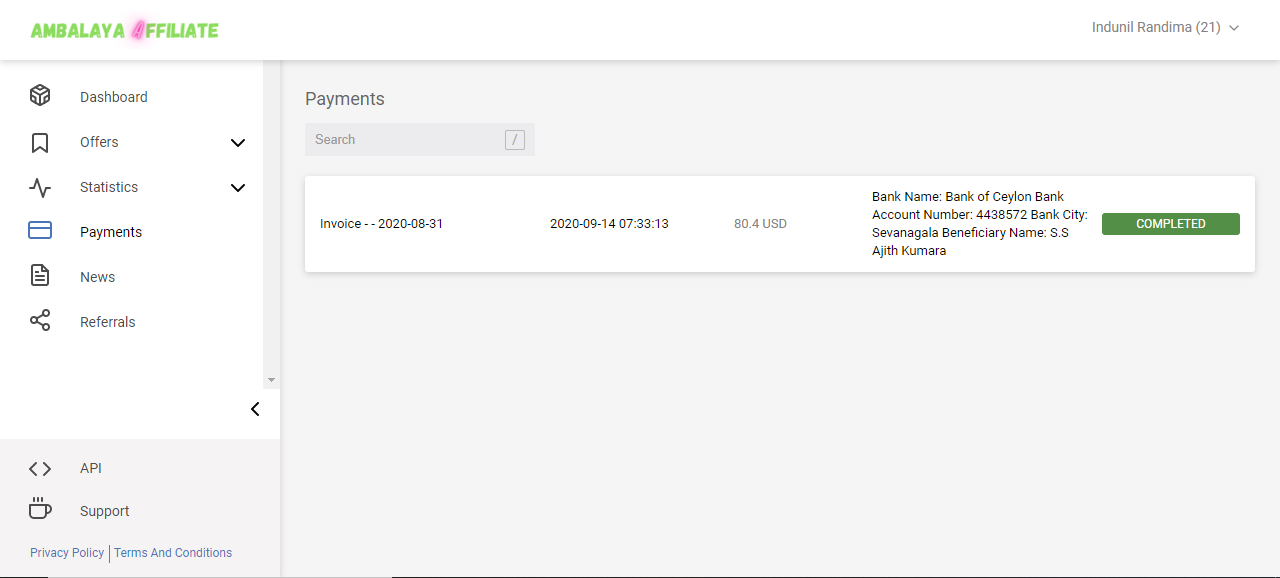The image depicts a computer monitor displaying an interface related to banking or invoicing. 

In the upper left corner, the screen is predominantly white, and it showcases the text "Ambalay Affiliate" with distinctive formatting: "Ambala" in green letters, "A" in pink and slightly tilted, and "FFILIATE" continuing again in green. 

To the right, it displays "Induniel Randima" with the number "21" and a downward caret inside parentheses.

On the left panel of the screen, which occupies less than the left corner and is also white, there are navigation options arranged in four rows:
1. A symbol followed by "Dashboard"
2. A symbol followed by "Offers"
3. A symbol followed by "Statistics"
4. A symbol followed by "Payments"
5. A symbol followed by "News"
6. A share symbol followed by "Referrals"

Below this panel, in a gray area, additional options are available:
- "API"
- "Support"

Further down, in a blue section, there are links to the "Privacy Policy" and "Terms and Conditions."

The majority of the screen to the right of this panel has a gray background. At the top, in gray text, it says "Payment." There is a search bar that reads "Search" but is currently empty.

Dominating the middle section of the screen is a white pane that stretches horizontally across, resembling an invoice detail. It reads:

- "Invoice -- 2020-08-31"
- Next column: "2020-09-14 07:33:13"
- Next column: "80.4 USD"
- Next column: "Bank Name: Bank of Ceylon Bank, Account Number: 4438572, Bank City: Galle, Beneficiary Name: SS Ajith Kumara"

In the final column, there is a green button with white letters stating "Completed."